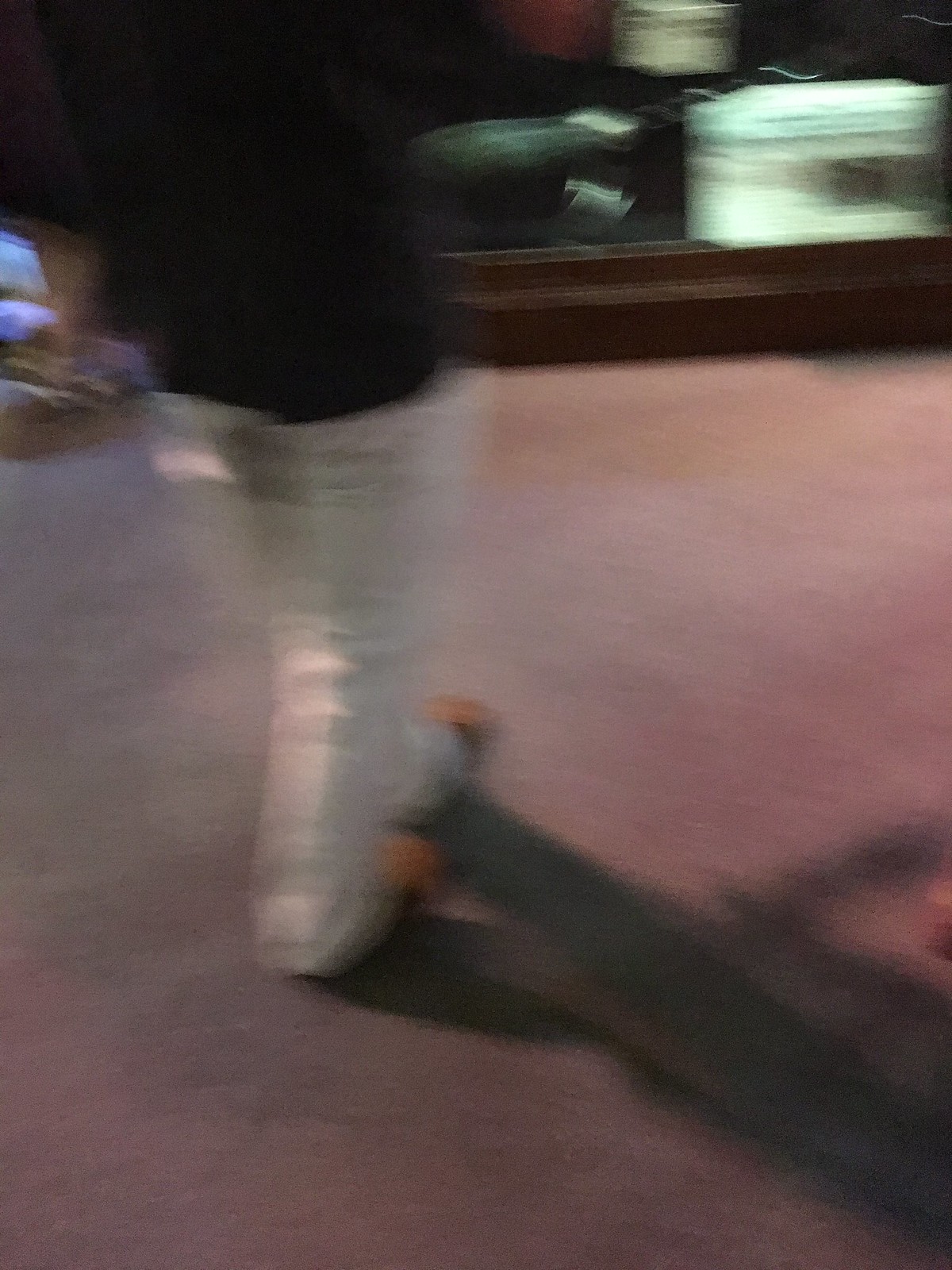A vertical, slightly blurry photo captures a person in a costume, viewed from behind. The individual is adorned with exceptionally high, bulky boots resembling thick bandages that extend well above their thighs. Visible beneath the costume are tips of shoes and black clothing. The scene is set on a pink-colored carpet, patterned with shadows. In the background, to the right, a TV console and screen are discernible, while to the left, a shiny item—possibly a speaker—can be seen on the shelf. In the upper left corner of the image, various indistinct items rest on the floor, including a cushion or pallet with vertical, illuminated white boxes. The person appears to be walking, placing one foot in front of the other.